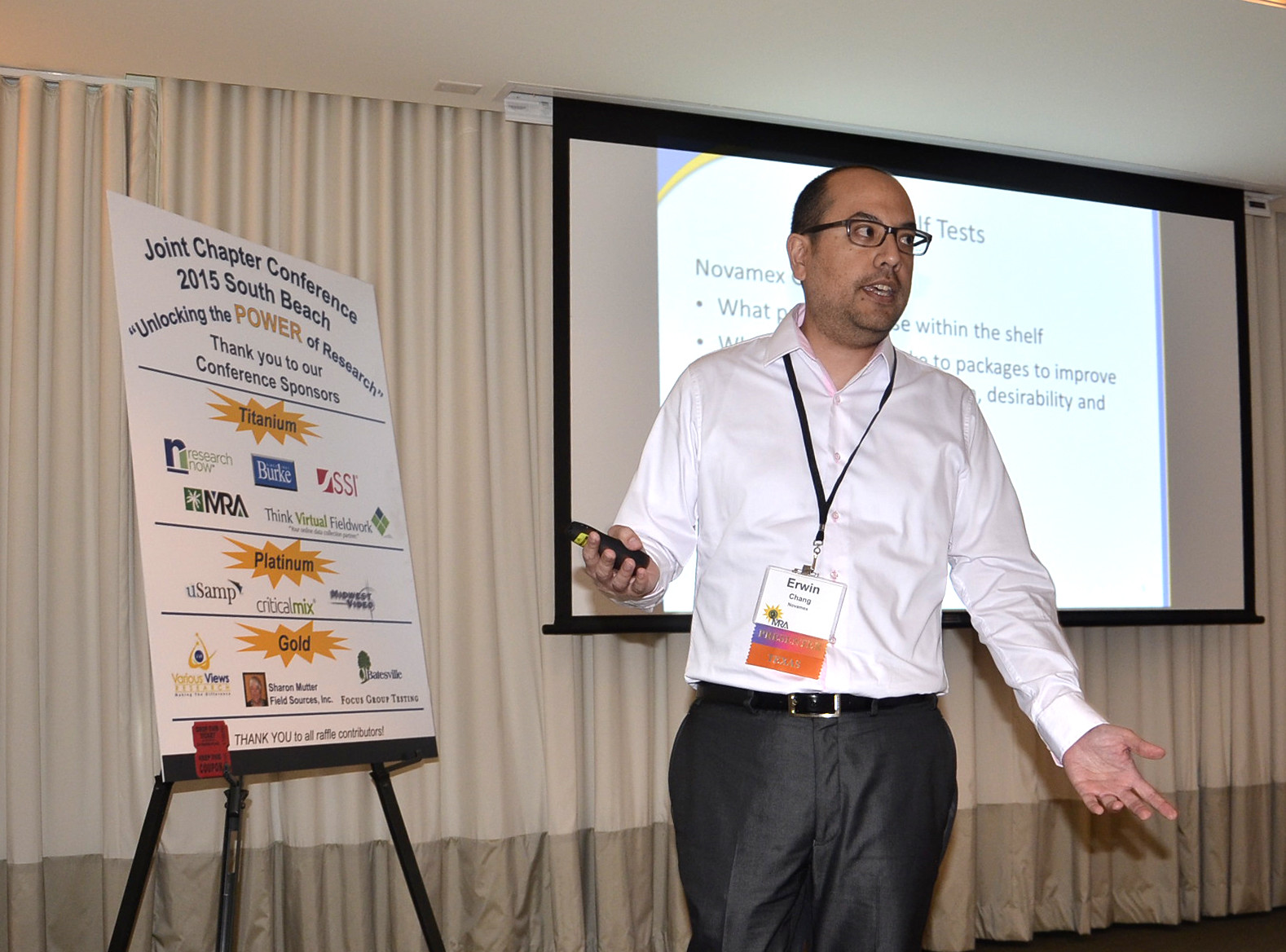In the rectangular photograph, a man named Erwin is delivering a presentation to a crowd, seemingly at a conference. He stands on a stage adorned with light cream curtains featuring a darker brown band at the bottom. The background includes a projection screen displaying a partially visible PowerPoint presentation, with discernible words such as "tests" and "Novamex." Erwin, dressed in a white dress shirt, black belt, and gray slacks, holds a projector clicker in one hand while speaking and engages the audience with the other hand gestured down by his hip. A name tag hangs around his neck, suspended by thin black cords. To his right, an easel setup displays a sign reading, "Joint Chapter Conference 2015 South Beach: Unlocking the Power of Research," alongside acknowledgments to various sponsors, symbolized by numerous logos and the labels "titanium," "platinum," and "gold."